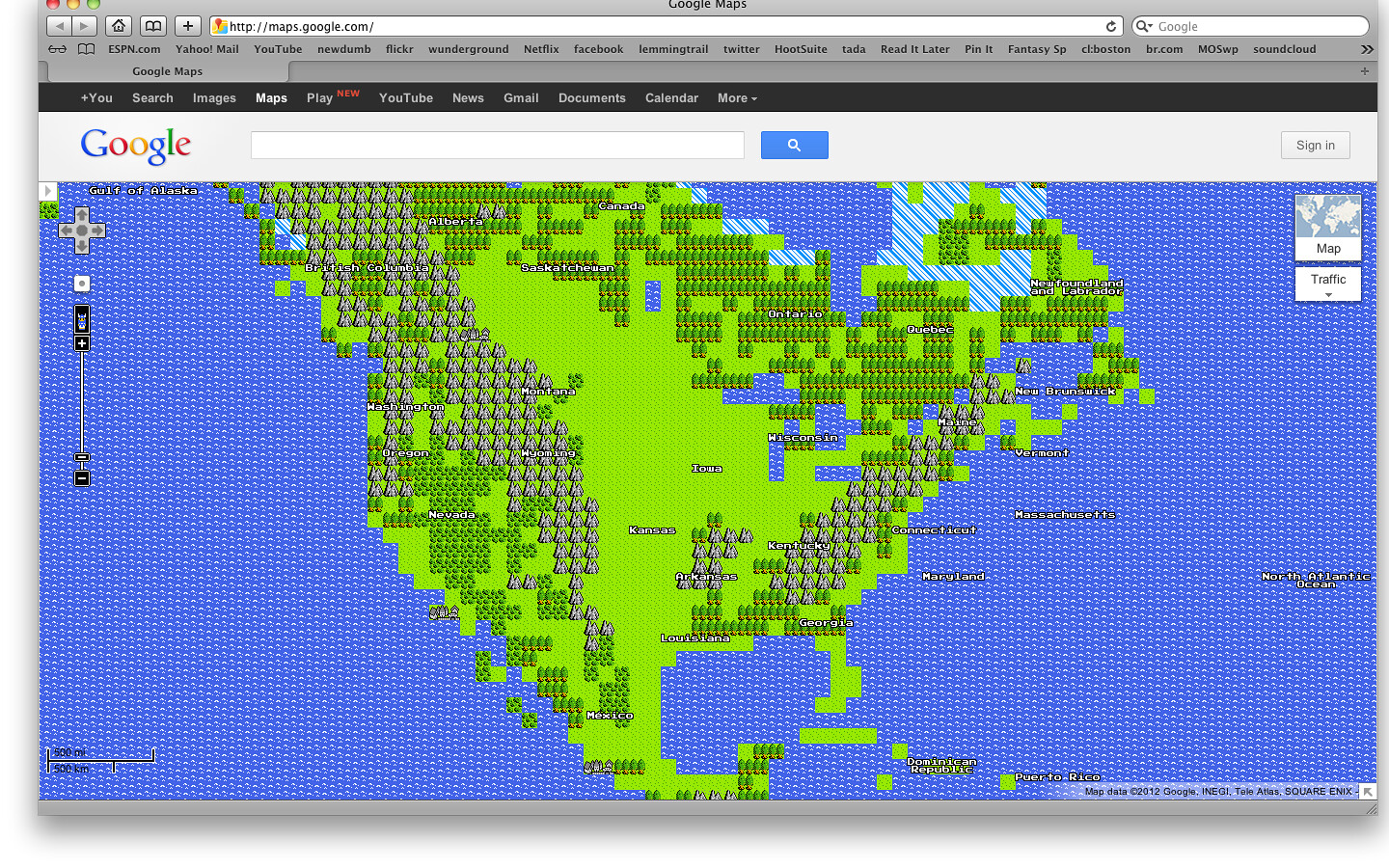This screen capture showcases a desktop computer display featuring a nostalgic, pixelated version of Google Maps accessed via the URL maps.google.com. The map predominantly highlights the United States and the surrounding Atlantic and Pacific Oceans. Despite the pixelation, some place names are discernible, although those over the oceanic regions, which include designations like the Mariana Trench and other notable underwater features, are somewhat blurred.

The United States map is depicted in a distinct grass green with darker green areas presumably representing forests, identifiable by their tree-like icons composed of dark green canopies and brown trunks. Urban areas or buildings are indicated with a stark gray coloring. Water bodies such as the Great Lakes and the Gulf of Mexico are rendered in blue, contributing to the geographical detail.

Several state names are faintly visible, with "Iowa" and "Michigan" partially distinguishable among others. Prominently, on the left side of the screen, a vertical zoom slider with plus and minus buttons allows for image magnification adjustment. This visual evokes a sense of the early days of digital cartography and the evolution of online map interfaces.